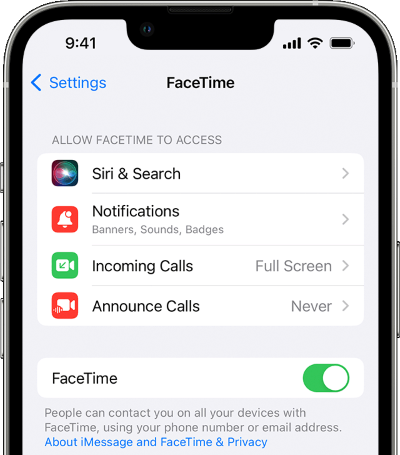Screenshot of an iPhone displaying the FaceTime settings page. The image shows only the upper half of the iPhone against a light gray background. The top section of the screen features a title "FaceTime," accompanied by a blue "Settings" label and a back button.

Beneath this, there is a section labeled "Allow FaceTime to Access," containing four options within a white window:
1. "Siri & Search"
2. "Notifications" (with additional info in small text: "Banners, Sounds, Badges," which means you can manage how to receive notifications)
3. "Incoming Calls," set to "Full Screen"
4. "Announce Calls," set to "Never"

Further down, on a white background, there's a bar labeled "FaceTime," which is toggled off. Below this, small text explains: "People can contact you on all your devices with FaceTime using your phone number or email address." A hyperlinked text at the bottom reads "About iMessage and FaceTime & Privacy."